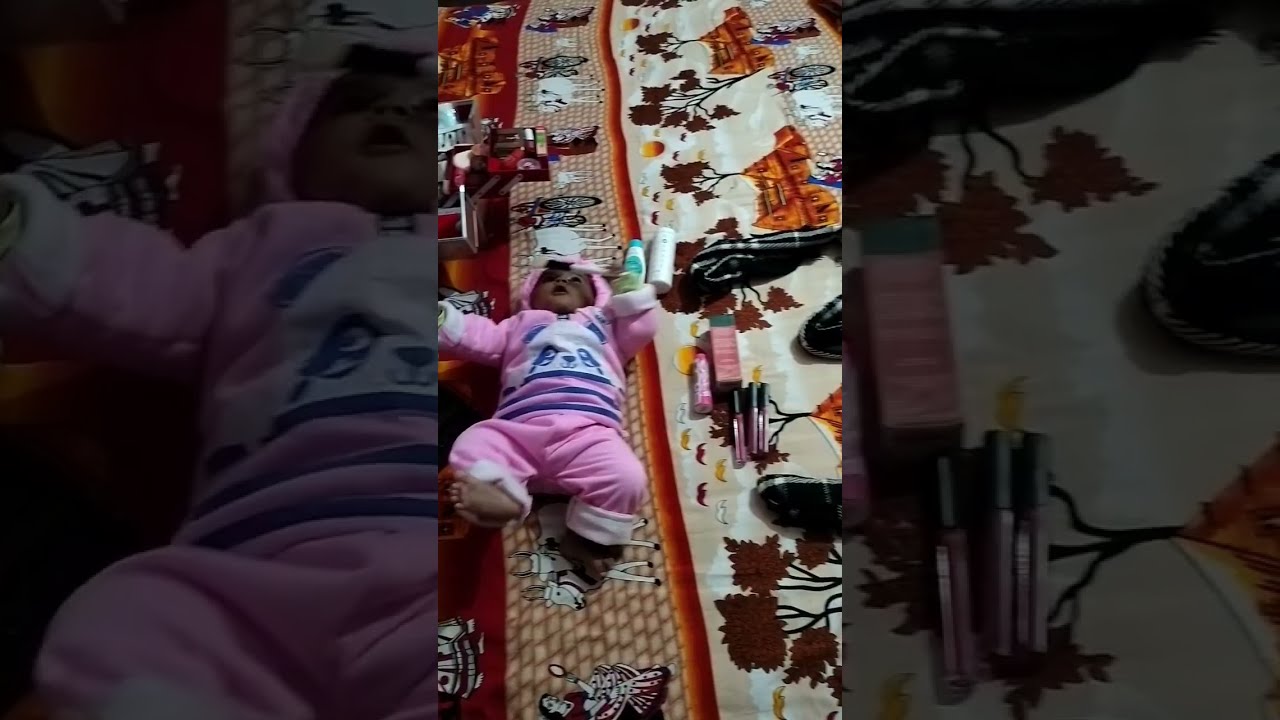The image is a detailed color photograph focusing on a dark-skinned baby lying on its back on a vibrant, multicolored carpet. The baby, possibly a girl, is dressed in a pink outfit featuring a panda bear design on the chest and includes a hood covering her head. The baby’s right foot, bare and pointed upward, contrasts with the soft material of the carpet. Her arms are outstretched, revealing two bottles—a white one and a white-and-teal one—just above her right shoulder. The background carpet is adorned with intricate designs of leaves, bicycles, animals, and elements resembling a brick walkway. Surrounding the baby are several personal care items, including three makeup cases with purple bases and black tops, and other grooming items such as plastic bottles in various colors. The photograph is inset within an enlarged, darkened portion of the same image, zooming in on specific details such as the baby’s position and the nearby items. The overall style of the photograph is representational realism, capturing the scene with clear, vibrant details and a dynamic, slightly blurred portrayal of the baby’s movements.